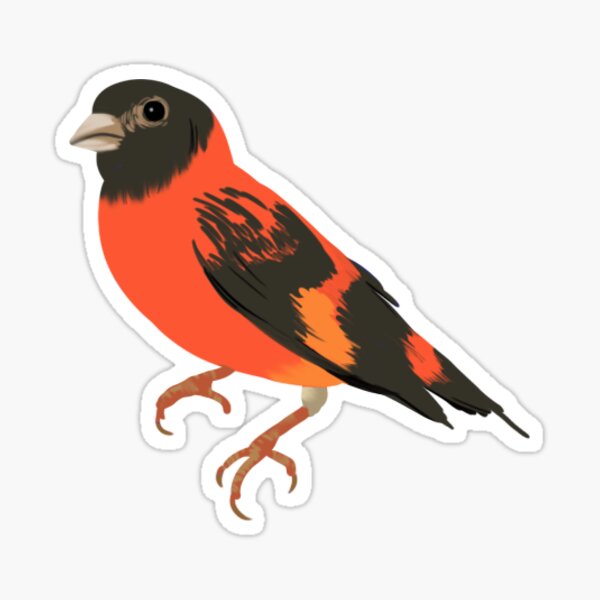The image showcases a cartoon-styled bird that resembles a red siskin. The bird is primarily red with black and red wings and a black head. It has a small, light brown beak that is thicker than it is long, giving it a distinctive appearance. The bird’s black eye, accented by a beige ring, appears focused to the left, and there is a white dot within the eye adding a beady effect. Its expression seems slightly frowning, possibly indicating it is upset. The bird has orange-colored feet with brown claws at the tips. The feathers feature speckled patterns with bright orange hues on the sides.

What stands out in this image is the sticker-like presentation of the bird. There is a white outline around the bird, followed by a gray shadow, which makes it look like it is placed on top of an eggshell white background. The true white border around the bird contrasts with the slightly off-white background, enhancing the sticker-like illusion.